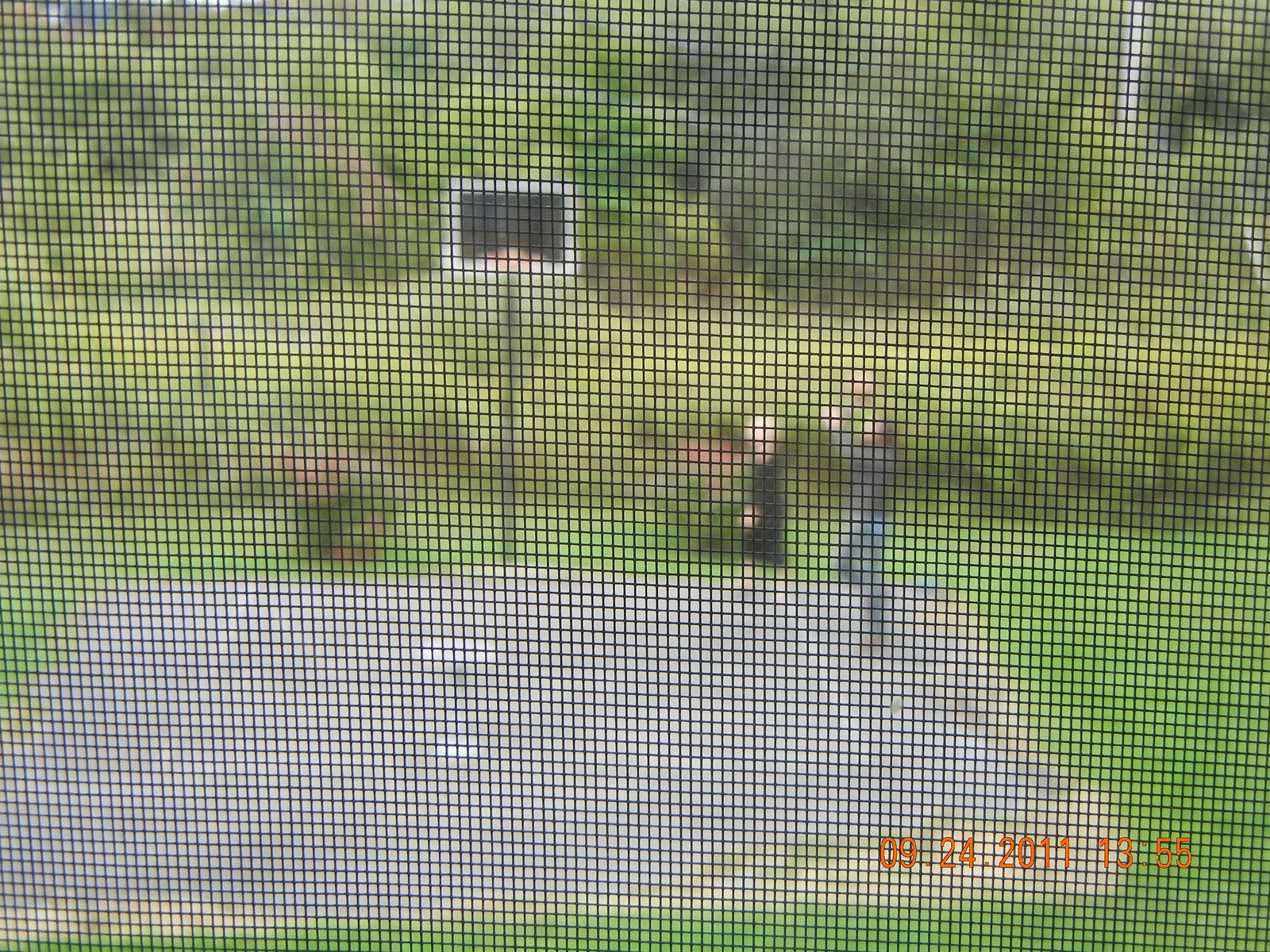The photograph, dated September 24, 2011, at 13:55, captures an outdoor basketball scene set in a lush green yard filled with trees. The image is taken through a screen, possibly a screen door or trampoline net, which unfortunately captures the screen’s mesh in focus rather than the play. The scene shows two individuals on the court; a man with brown hair dressed in a green shirt and jeans, standing on one leg and appearing ready to take a shot from a side line. Opposite him stands a child, possibly a boy, with blonde hair, wearing a black outfit. The child is seemingly poised to catch or intercept the ball. They are playing on a dark gray court with a black basketball hoop and backboard mounted on a pole. The photo emits the casual and energetic vibe of a pickup game in a backyard setting.